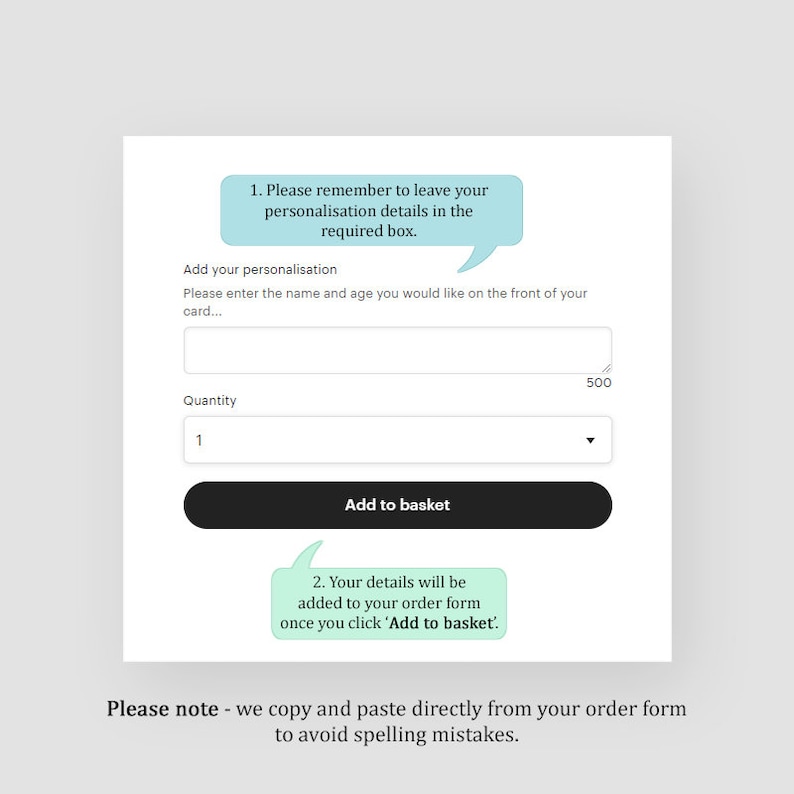The image displays a website interface for customizing and purchasing a personalized item. The layout features a gray box containing a white box. At the top, a turquoise message bubble with a line extending downward is labeled with "1" and instructs users: "Please remember to leave your personalization details in the required box." Below this, text prompts users to "Add your personalization: Please enter the name and age you would like on the front of your card," providing a dedicated space for input.

Following the personalization box is a dropdown menu where users can select the quantity of their desired items. Directly beneath this is a prominent black button labeled "Add to Basket" in white text, ensuring high visibility. 

Further down, another turquoise message bubble marked with "2" informs users: "Your details will be added to your order form once you click add to basket." Additional text in bold black warns: "Please note, we copy and paste directly from your order form to avoid spelling mistakes." This notice clarifies that the responsibility for any errors in the provided information lies with the user, as the details are directly transferred from the input form to the final product.